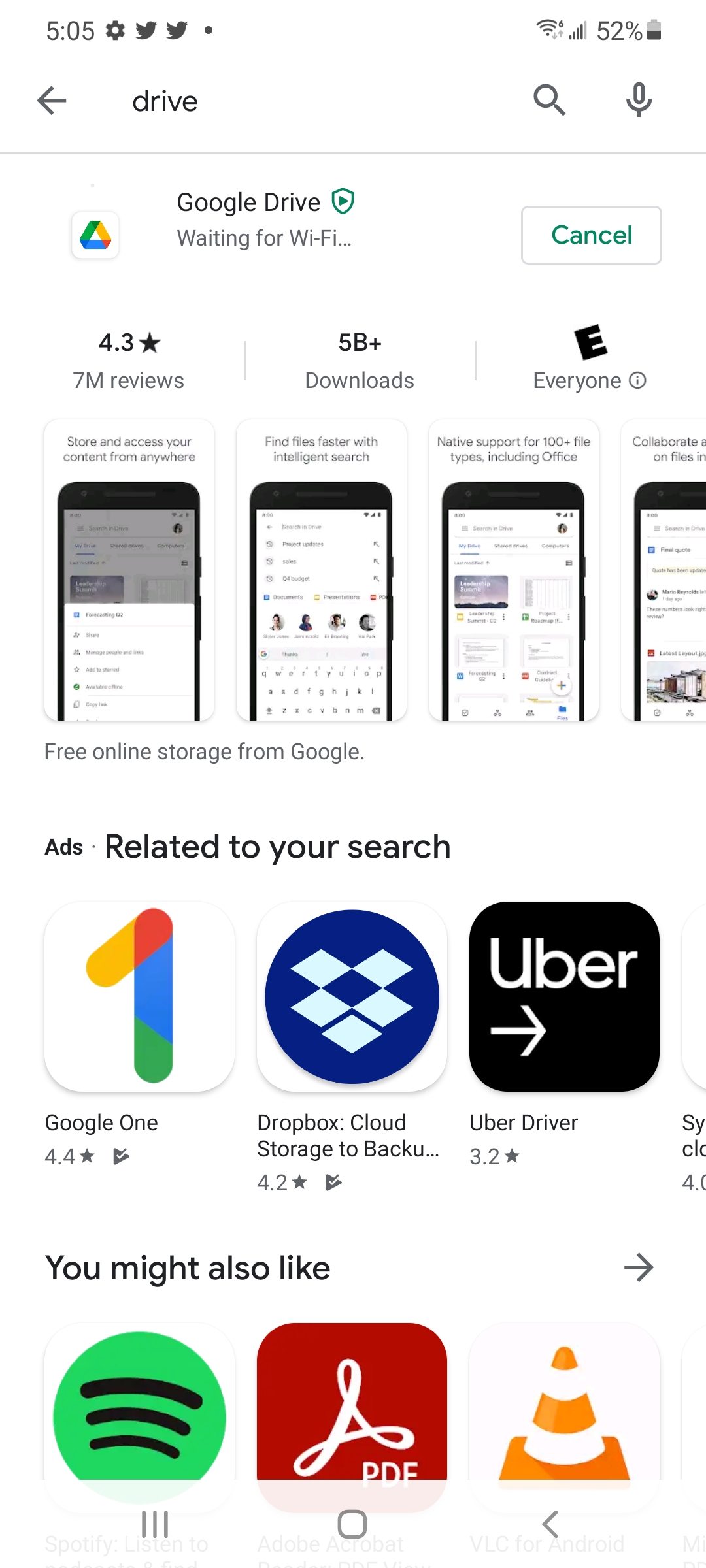The image is a screenshot from a smartphone. In the top left corner, the time is displayed as 5:05, accompanied by a small gear icon, two Twitter icons, and a very small dot. On the top right, the Wi-Fi signal indicator shows full bars, and the battery level is at 52%. In the search bar, the word "Drive" is entered, yielding Google Drive as the search result, alongside related ads. Featured icons include Google One, Dropbox cloud storage for backup, and Uber Driver. There are additional icons at the bottom which are partially cut off. Near the top section of the screen, there are three visible images of phones with screenshots. The first screenshot promotes storing and accessing content from anywhere, the second highlights finding files faster with intelligent search, and the third mentions native support for over 100 file types, including Office. The fourth image's content is partially cropped and not fully visible.